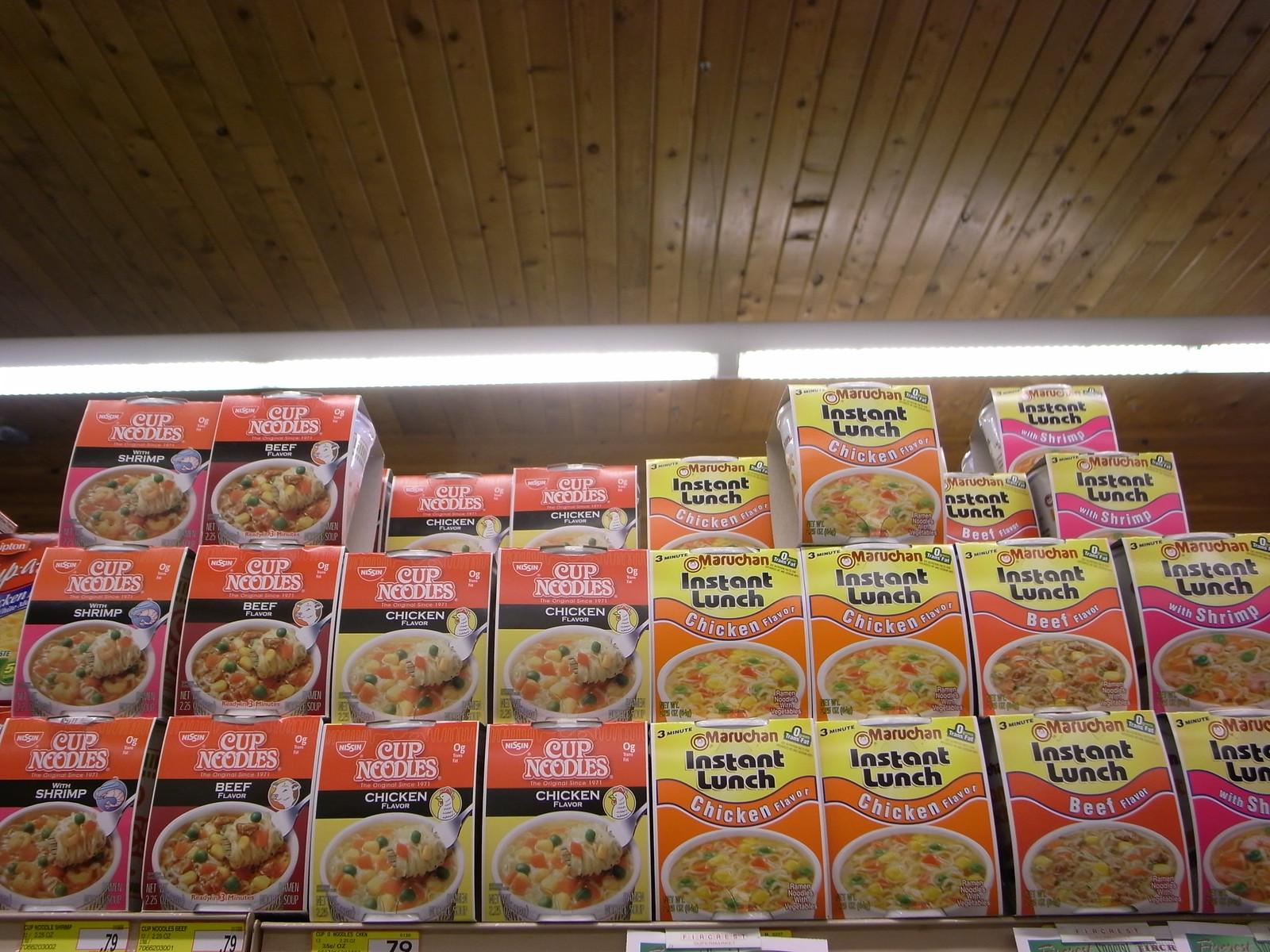The photograph captures a detailed scene inside a store, focusing on shelves stocked with various noodle products beneath a timber wood ceiling with visible dark knots and circles. Rectangular, horizontal white fluorescent lights hang from the ceiling, illuminating the scene. On the left side of the shelf, boxes of “Cup Noodles” are stacked, identified by their orange-topped labels with white writing. Below this, a black rectangle displays the flavor "Chicken," accompanied by an image of a white bowl filled with chicken, peas, and carrots on a yellow background. Next to these, other boxes showcase "Beef" and "Shrimp" flavors, distinguishable by pink accents.

On the right side of the image, the products shift to “Maruchan Instant Lunch,” featuring rectangular packaging with a yellow top that says “Instant Lunch” in black, an orange ribbon beneath it, and the flavor indicated in the lower half. The chicken flavor packaging also displays a bowl of noodles in yellow broth with peas and carrots. This side contains various flavors, including "Chicken," "Beef," and "Shrimp," arranged in neat rows. A yellow price tag in the lower section of the image reads “.79” in black on a white rectangle. Flavors and brands are systematically organized, enhancing the visual appeal and clarity of product variety and pricing within the store aisle.